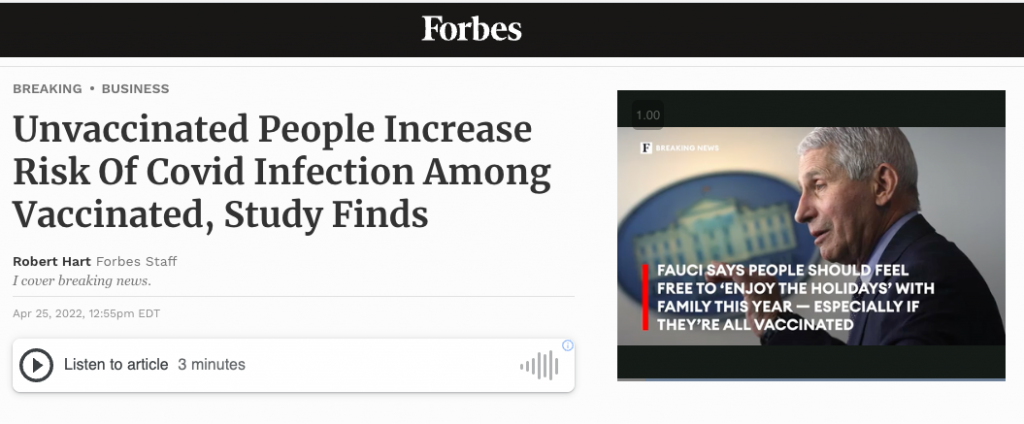The image contains a prominent black rectangular banner at the top with the word "Forbes" in white text, centered. Below this banner, there are two labels on the left: "Breaking" and "Business". The main headline, written in black text, reads: "Unvaccinated people increase risk of COVID infection among vaccinated, study finds." 

Directly under the headline, the author's name "Robert Hart" appears, with "Forbes Staff" noted to the right in light gray text, followed by the author's description, "I cover breaking news." A thin, gray horizontal line separates this information from the time and date "April 25th 2022, 12:56 PM EDT" below. 

To the right, there is a small circle icon containing a right-pointing arrow, which indicates, "Listen to article, 3 minutes".

Adjacent to this section is an image of Dr. Anthony Fauci, positioned to the right and shown in a profile view. Dr. Fauci stands in front of a backdrop featuring the Capitol Building. He is dressed in a navy blue suit jacket over a blue collared shirt, and he has short gray hair. Below Dr. Fauci's image, a quotation reads: "Fauci says people should feel free to enjoy the holidays with family this year, especially if they’re all vaccinated." A short vertical red line is placed beside this quotation.